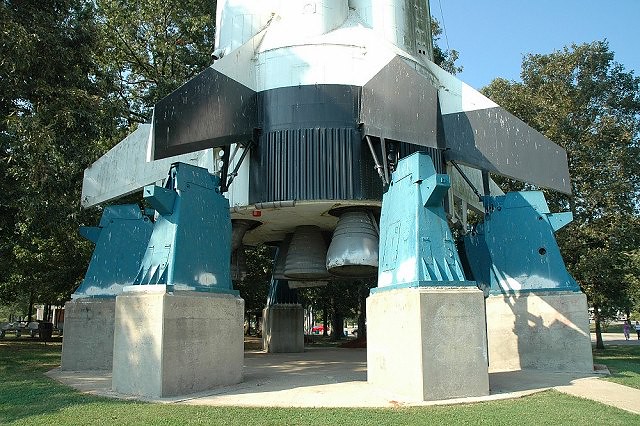The image depicts the bottom of a rocket resting on five concrete blocks within a large concrete circle, surrounded by a flat, grassy field. The scene is set outdoors on a sunny day, with the sun casting shadows from the right. The rocket's tail, featuring a black and white section with corrugated details in the middle, is prominently centered in the image. Below the tail, blue pylons support the rocket boosters, which consists of several silver-colored cylinders. The display is augmented by green trees on either side, framing the backdrop of the lush, verdant surroundings. The sky is a clear blue, adding to the vividness of the setting.

Note: Although the second description mentions a sidewalk and additional elements like buildings and vehicles, these aspects were not incorporated in the final detailed caption to avoid conflicts with the overlapping details provided in the other descriptions.